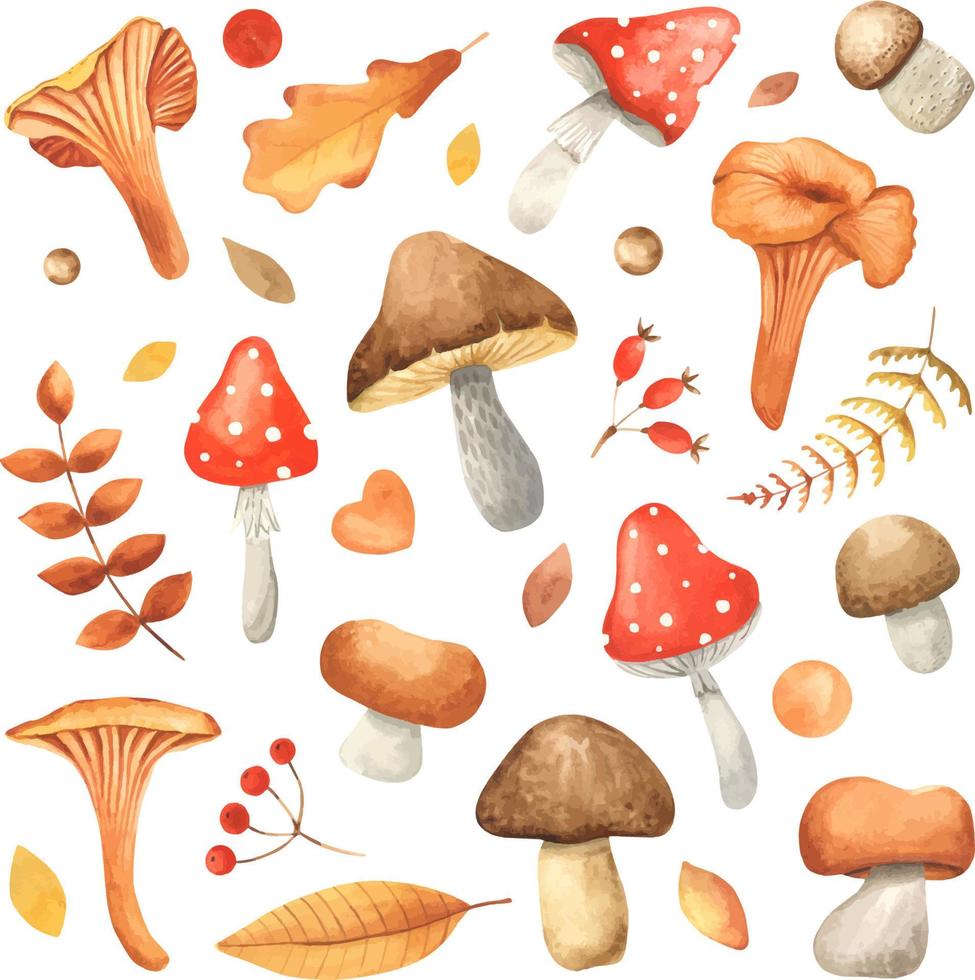The image is a detailed, hand-drawn illustration set against a white background, featuring a diverse array of organic elements you might encounter on a nature hike. The primary focus is an assortment of mushrooms, with around a dozen different varieties depicted. These include the iconic red mushrooms with white dots often seen in cartoons, as well as more realistic species with white stems and brown tops. Some mushrooms are thick with rounded caps, while others are thin-stemmed or have more unusual shapes like triangular and rectangular caps. Interspersed among the mushrooms are various leaves, branches, and what appear to be clusters of berries or fruits, including radish-like and cherry-like formations. The scene also includes depictions of sweet potatoes, individual leaves, and possibly wheat or other seeds. The drawing evokes the look and feel of vintage wallpaper, with a rich color palette including reds, browns, and whites, but without any textual elements present.